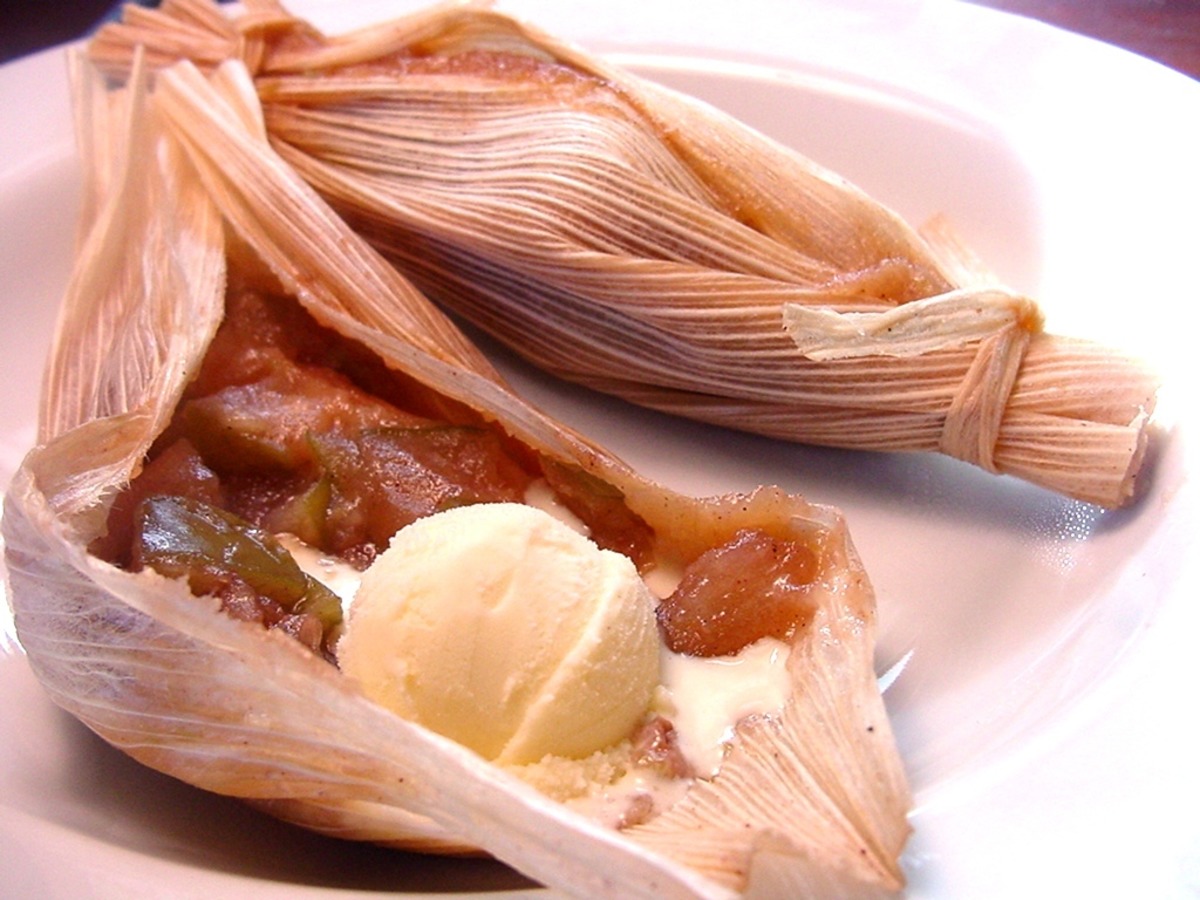The image depicts a well-lit, restaurant-style setting featuring two food items presented on a wide, white plate. These items resemble tamales, wrapped in corn husks, with one being closed and tied at both ends, while the other is partially unwrapped to reveal its filling. The filling appears to include some pieces of fat, potential green vegetables, and possibly some form of matzah or other grain. It's unclear if there's meat among the ingredients. Accompanying these food items is a generous scoop of vanilla ice cream, which is slightly melted and pooling around the base of the tamales, enhancing the dish's rich textures and flavors. The overall tone of the image is tinged with a yellowish hue, possibly due to the restaurant's lighting.